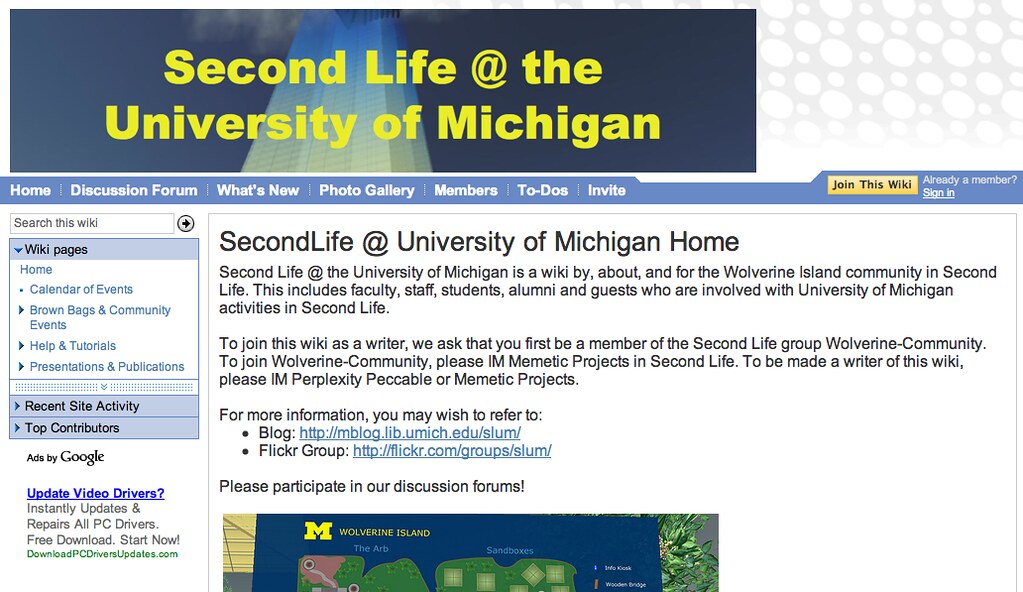The image captures the homepage of a website affiliated with the University of Michigan. The layout features a white backdrop adorned with a subtle gray pattern. Dominating the top of the page is a dark blue banner displaying the text "Second Life at the University of Michigan" in bright yellow lettering. This banner is underlaid with an abstract design reminiscent of a flower top. 

Directly beneath this, the main content area begins, featuring a mauve-blue navigation bar. The navigation menu, styled in white font, includes the following buttons: Home, Discussion Forum, What's New, Photo Gallery, Members, To-dos, and Invite. On the far right of this navigation bar, there are options to "Join this Wiki" in a yellow button and "Already a Member" followed by a "Sign In" link in white.

On the left-hand column, the website contains a search function labeled "Search This" and a section titled "Wiki Pages," highlighted in a pale lilac color. Bold white text under this header lists several hyperlinks: Home page, Calendar of Events, Brown Bags and Community Events, Help and Tutorials, and Presentations and Publications. Further down, two additional mauve buttons are labeled "Recent Site Activity" and "Top Contributors," followed by a section featuring Google advertisements. The specific ad visible is titled "Update Video Drivers."

The main body of the page, situated to the right of the left-hand column, begins with a prominent headline stating "Second Life at University of Michigan Home." Below this, a detailed description reads, "Second Life at the University of Michigan is a wiki by, about, and for the Wolverine Island community in Second Life. This includes faculty, staff, students, alumni, and guests who are involved with University of Michigan’s activities in Second Life." It further notes the requirements for joining the wiki as a writer, urging members to join the Second Life group Wolverine community, and provides contact information for Mimetic Projects and Perplexity Packable.

Additionally, the website offers links for further information through two clickable bullet points leading to a blog (http://lmblog.lib.umich.edu/slum) and a Flickr group (http://flickr.com/groups/slum). The page invites visitors to participate in discussion forums, and the lower section hints at an image partially visible at the bottom.